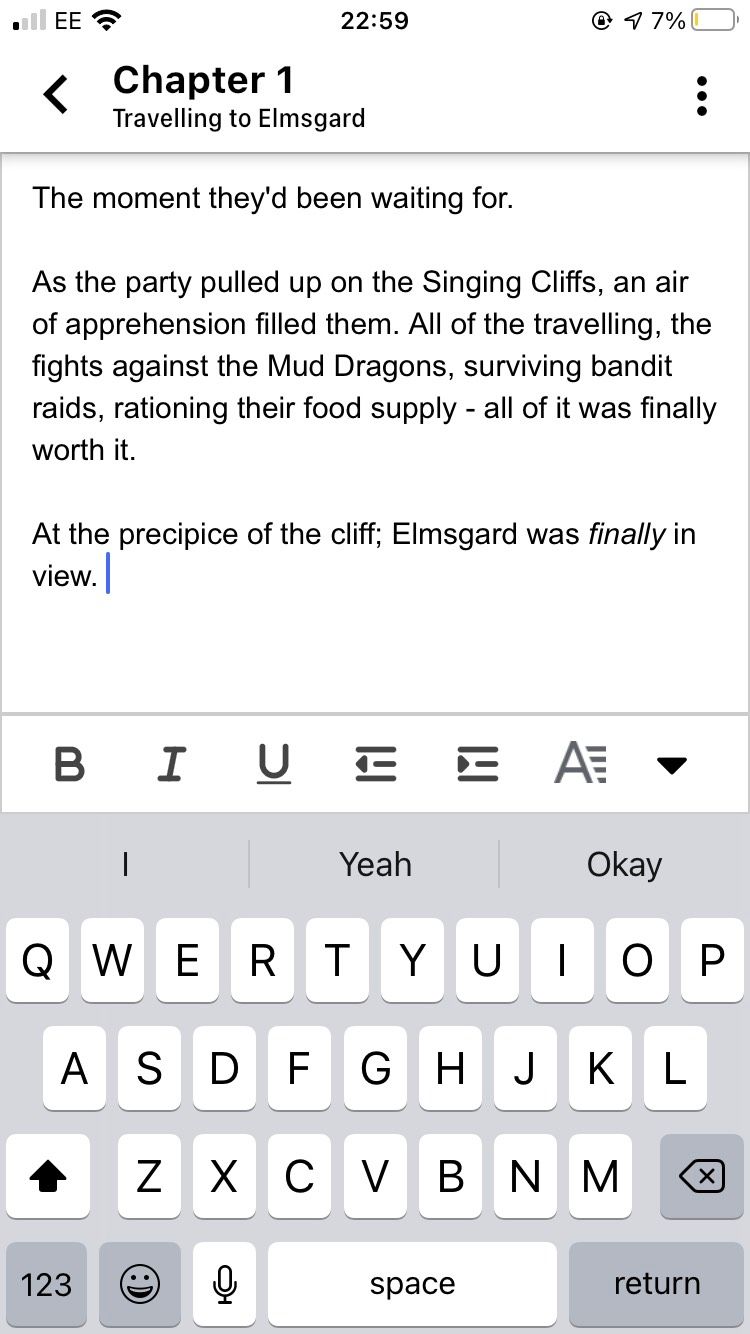A cell phone screenshot is displayed with various elements. In the top left corner, a signal strength indicator shows one bar, accompanied by the letters "EE" in capital letters. Next to it, the Wi-Fi signal strength is displayed as full. At the middle top, the time is indicated as 22:59. In the top right corner, there is a lock icon in a circle, an arrow pointing to the top right, and the battery level at 7%.

Below these indicators, an arrow pointing to the left is followed by the text "Chapter 1" in bold. The next line reads "Traveling to Elmsgard." On the far right, three vertical dots are visible. 

Beneath this, text reads: "The moment they’ve been waiting for as the party pulled up on the singing cliffs. An air of apprehension filled them all. The traveling, the fights against mud dragons, surviving bandit raids, rationing their food supply—all of it was finally worth it." On the following line, "At the presence of the cliffs, Elmsgard was finally in view," with "finally" italicized.

Further down, formatting options are shown: the letters "B," "I," and "U" with an underline, followed by style formats. The words "I," "Yeah," and "Okay" appear below this, and finally, at the very bottom, a QWERTY keyboard is visible.